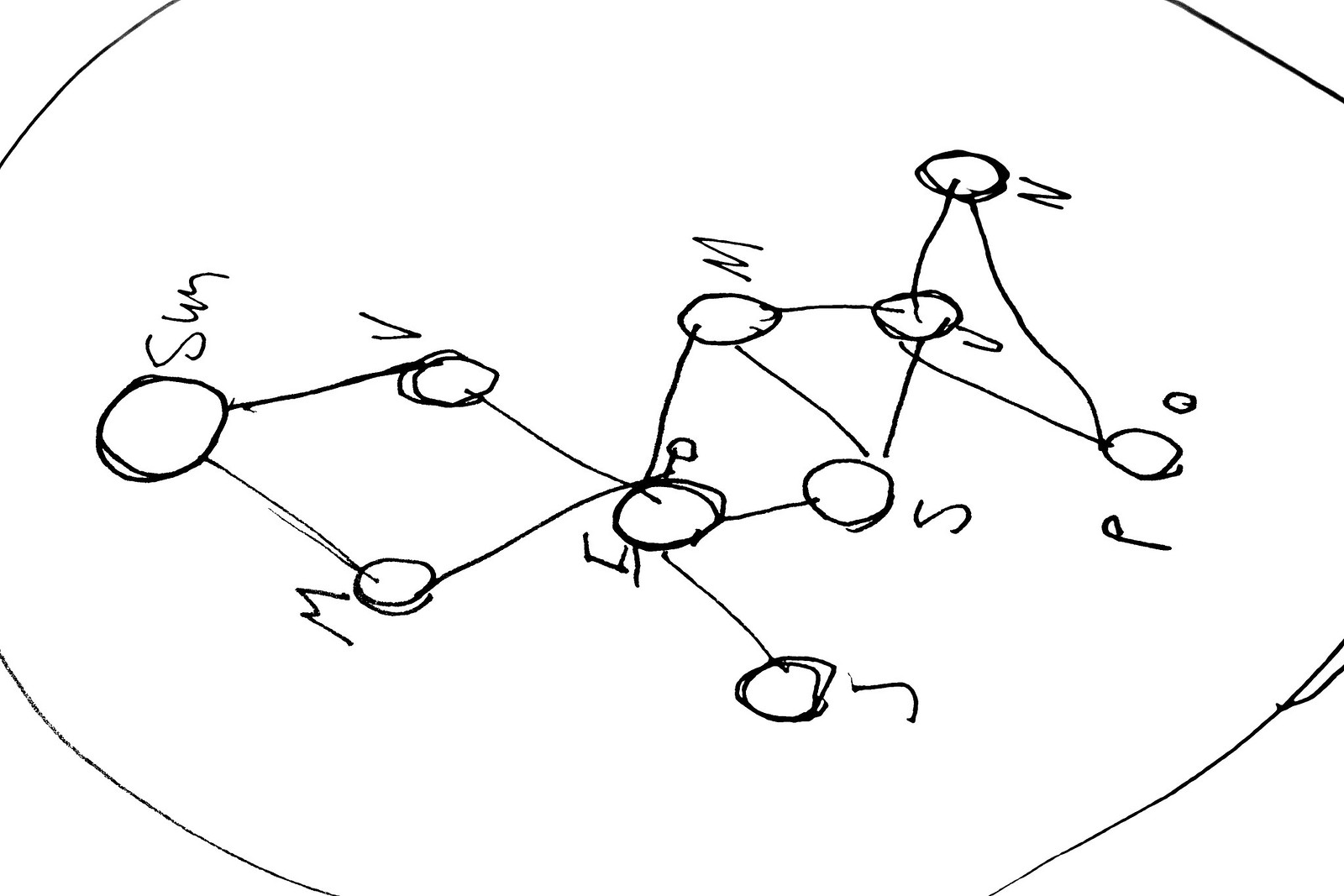This is an image of a drawing with geometric shapes and labels, captured on a piece of paper. Each of the four corners of the paper features a triangle, with its base aligned parallel to the sides of the paper and its apex pointing towards the center.

At the center of the drawing is a prominent circle labeled "Sun." Two lines extend from the Sun in opposite directions, each connecting to smaller circles labeled "M" and "V." These secondary circles meet at another central circle, which contains an indistinguishable letter that forms a complex hub of connections.

From this central circle with the indeterminate letter, the following lines and connections emanate:
- One line leads to a circle labeled "J."
- Another line leads to a circle labeled "S."
- Another line leads to a smaller circle also labeled "M," which further connects to the "S" circle and an additional unidentified circle.

The first central circle with the unknown letter has five lines extending out to various circles, creating a web of connections. The second unidentified circle has four lines branching out, with the bottom two lines leading to circles labeled "P" and "N." Adjacent to the "P" circle is an even smaller circle, similarly mirrored by a small circle next to the first unknown letter circle.

Overall, the drawing consists of a sun-centered network of interconnected circles and lines, with detailed annotations implying specific relationships and hierarchies among the labeled elements.